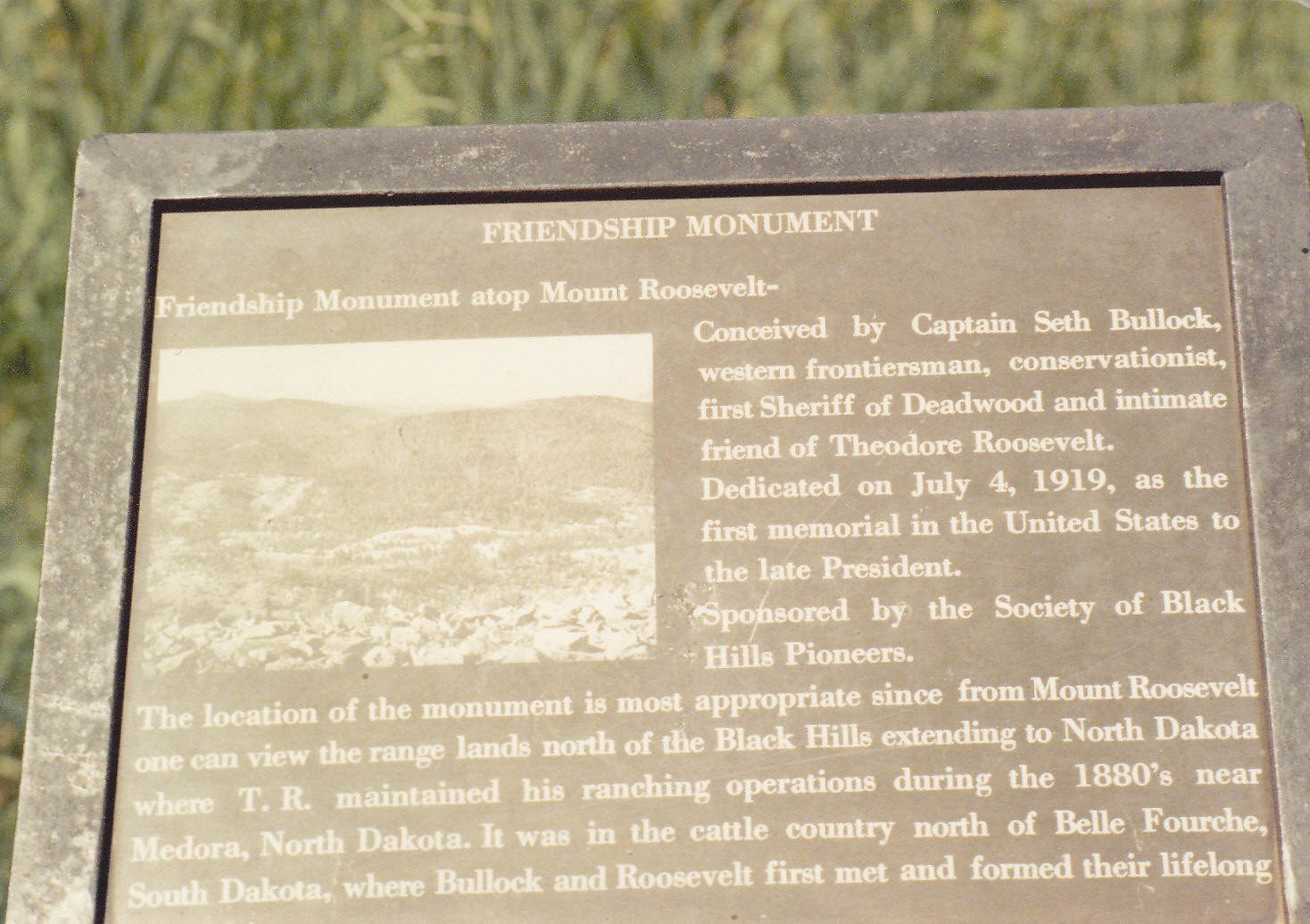The image depicts an outdoor scene with a slightly blurry background featuring grass, setting the stage for a weathered, gray-green plaque. This plaque, bearing signs of wear, prominently displays its message in all-capital white print. Centered at the top it reads "Friendship Monument," followed by "Friendship Monument atop Mount Roosevelt." To the left side of the plaque is a shadowy, indistinct picture. Adjacent to this image, the text continues: "Conceived by Captain Seth Bullock, Western frontiersman, conservationist, first sheriff of Deadwood, and intimate friend of Theodore Roosevelt. Dedicated on July 4th, 1919 as the first memorial in the United States to the late president. Sponsored by the Society of Black Hills Pioneers." Further description includes a truncated historical note indicating that the monument's location is significant, providing views of the rangelands north of the Black Hills extending to North Dakota, where Theodore Roosevelt ranched during the 1880s near Medora, North Dakota. It briefly mentions that Bullock and Roosevelt met and formed a lifelong friendship in the cattle country north of Belle Fourche, South Dakota.